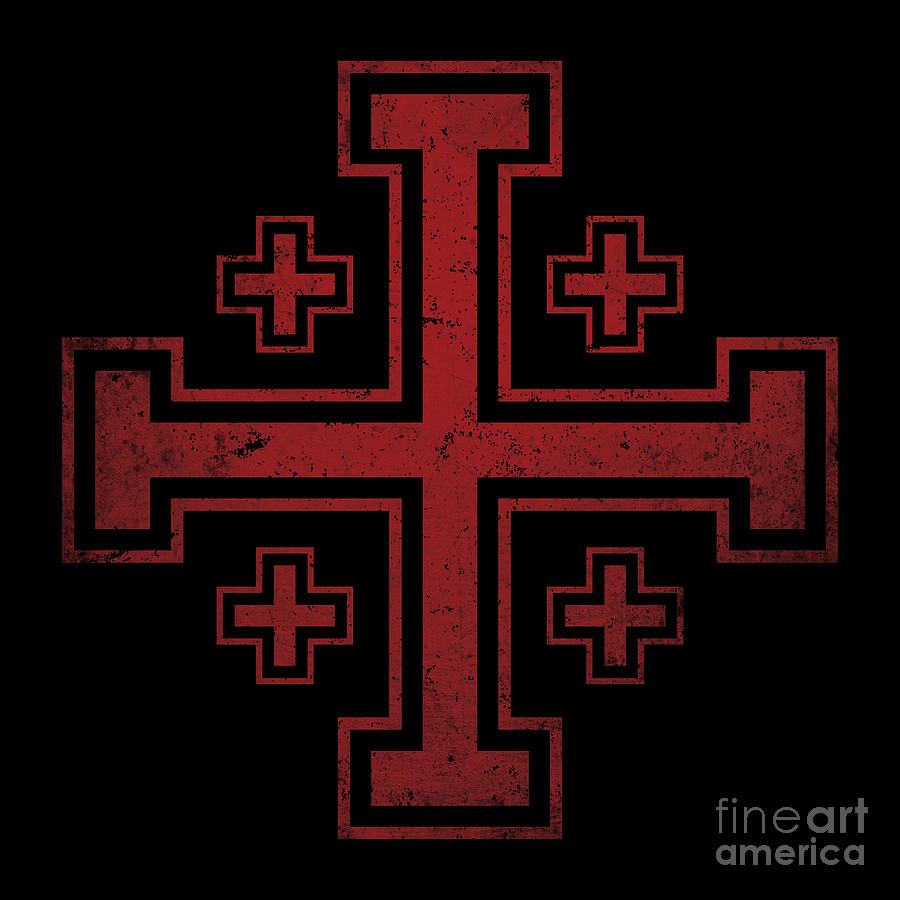The image is a digital design featuring a black background with a prominent central red cross, resembling a plus sign with small foot-like protrusions at the end of each arm. Surrounding this central cross, in each of its four internal corners, are four smaller red crosses. These smaller crosses are positioned in the top left, top right, bottom left, and bottom right quadrants of the larger cross. All the crosses exhibit a grungy, speckled black and red appearance, giving them a worn, textured look. The red graphics have a black outline and an additional red outline. The photo is watermarked in the bottom right corner with the label "Fine Art America," ensuring credit to the source. The stark contrast between the vivid red crosses and the deep black background creates a striking visual effect.